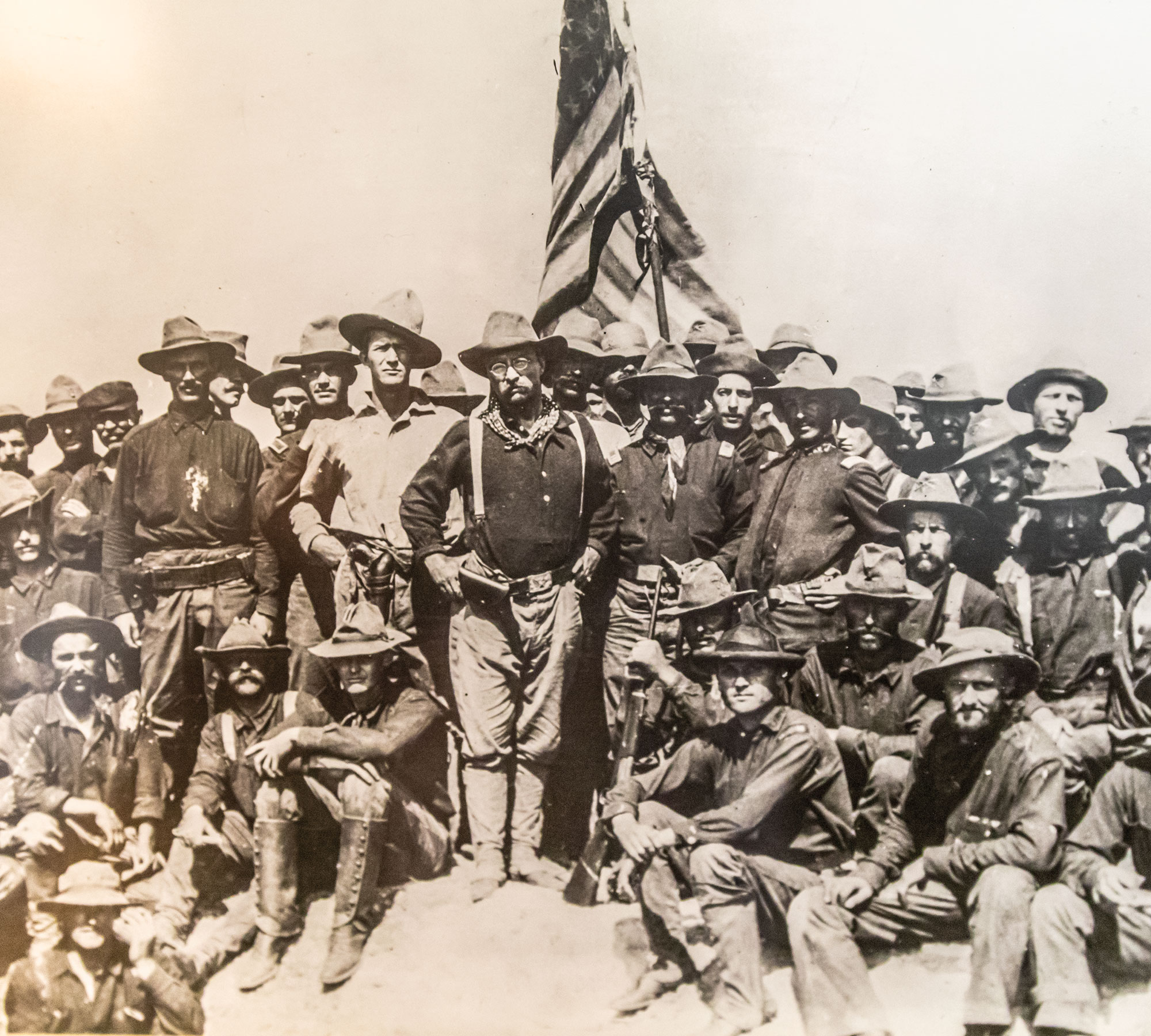This worn, sepia-toned photograph depicts a group of men standing in formation, facing the camera. Positioned centrally behind them is the American flag. The men, dressed uniformly in long-sleeve shirts, jeans, and leather boots extending to their knees, also sport floppy cowboy hats. The ground beneath them is barren, suggesting a sunlit, arid environment. In the center stands a distinguished figure with round glasses and a mustache, unmistakably Theodore Roosevelt. He wears a bandana around his neck and rests his hands on his trousers. Most of the men in the photograph, possibly gunmen or military personnel, are equipped with visible sidearm holsters, contributing to the image's historic war-time or Western Frontier ambiance.